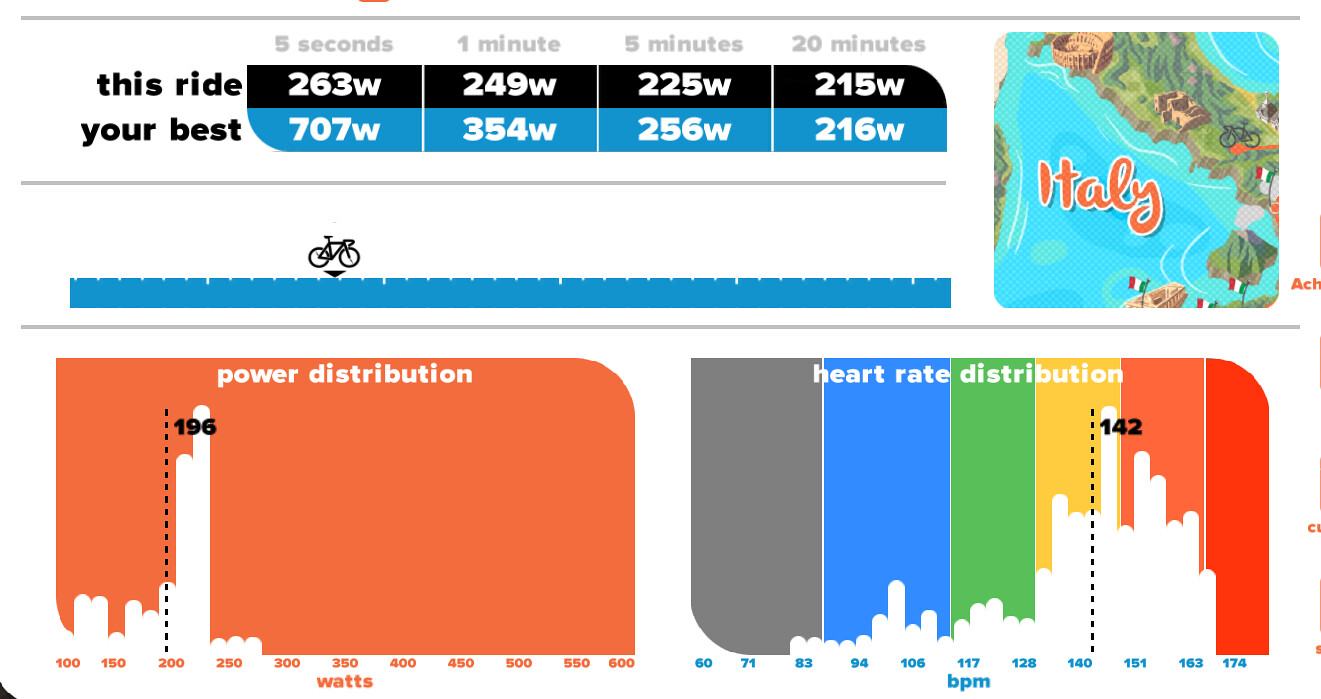The image is a detailed graphic depicting a cyclist's performance statistics, comprising multiple sections and visual elements. At the top left, the heading "This Ride" appears in black font, with black boxes next to it displaying power outputs for various time intervals: 5 seconds at 263 W, 1 minute at 249 W, 5 minutes at 225 W, and 20 minutes at 215 W. Directly below, labeled "Your Best" in black font, are blue boxes showing past best power outputs: 5 seconds at 707 W, 1 minute at 354 W, 5 minutes at 256 W, and 20 minutes at 216 W.

To the right of these statistics is a graphic featuring a bicycle traveling along what resembles a ruler, indicating the distance covered. Next to this is an illustrative representation of Italy, including a body of water and a green road, perhaps suggesting a thematic background of an app or location.

Beneath this section, there are two more graphs. The first is an orange power distribution graph with white segments and numerical breakdowns. The second is a colorful heart rate distribution graph located at the bottom right, displaying a vibrant spectrum of grey, blue, green, yellow, orange, and red. Together, these elements comprehensively visualize the cyclist's performance in terms of power output and heart rate distribution across various time intervals.